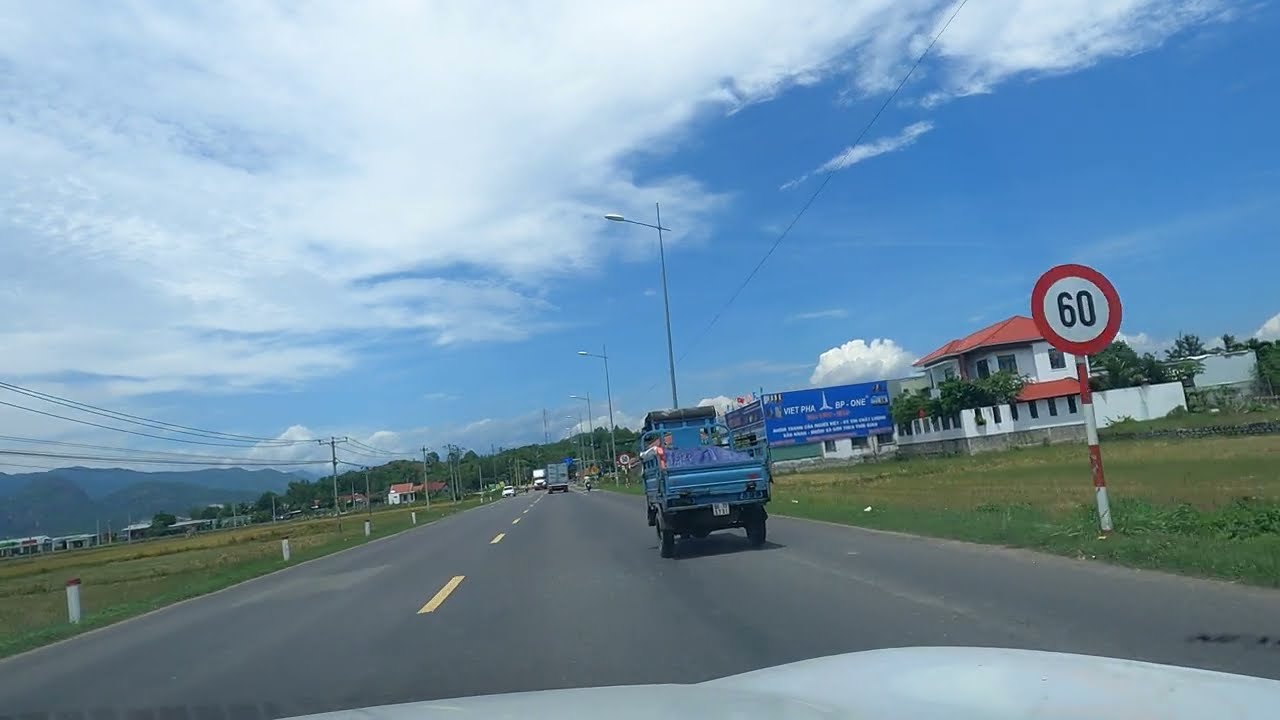In this color photograph taken from a vehicle's dash cam looking ahead on a highway, the viewpoint reveals a two-lane asphalt road with a yellow striped line down the middle, showing some missing sections. A speed limit sign on the right side of the road, mounted on a red and white pole, displays a black "60" inside a red circle on a white background. Ahead, a blue pickup truck with a black bumper and a white license plate is seen, while further down, a semi-truck with gray back doors is straight ahead, and another white truck is coming from the opposite direction on the left. Power lines and poles run along the left side of the road, where you'll also find safety barriers in white with red tops. On the right side, there's a two-story white building with an orange arched roof, partially covered by climbing vegetation reaching towards the second floor. Beside it, a white billboard and another blue billboard with white lettering stand against a backdrop of dense, distant trees. Overhead, the sky stretches out with its right side mostly clear and blue, and the left side dotted with light clouds. Metal streetlights line the right side of the road, directly over the street. In the vicinity, expanses of farmland and small mountains appear, enhancing the scenic but semi-urban setting.